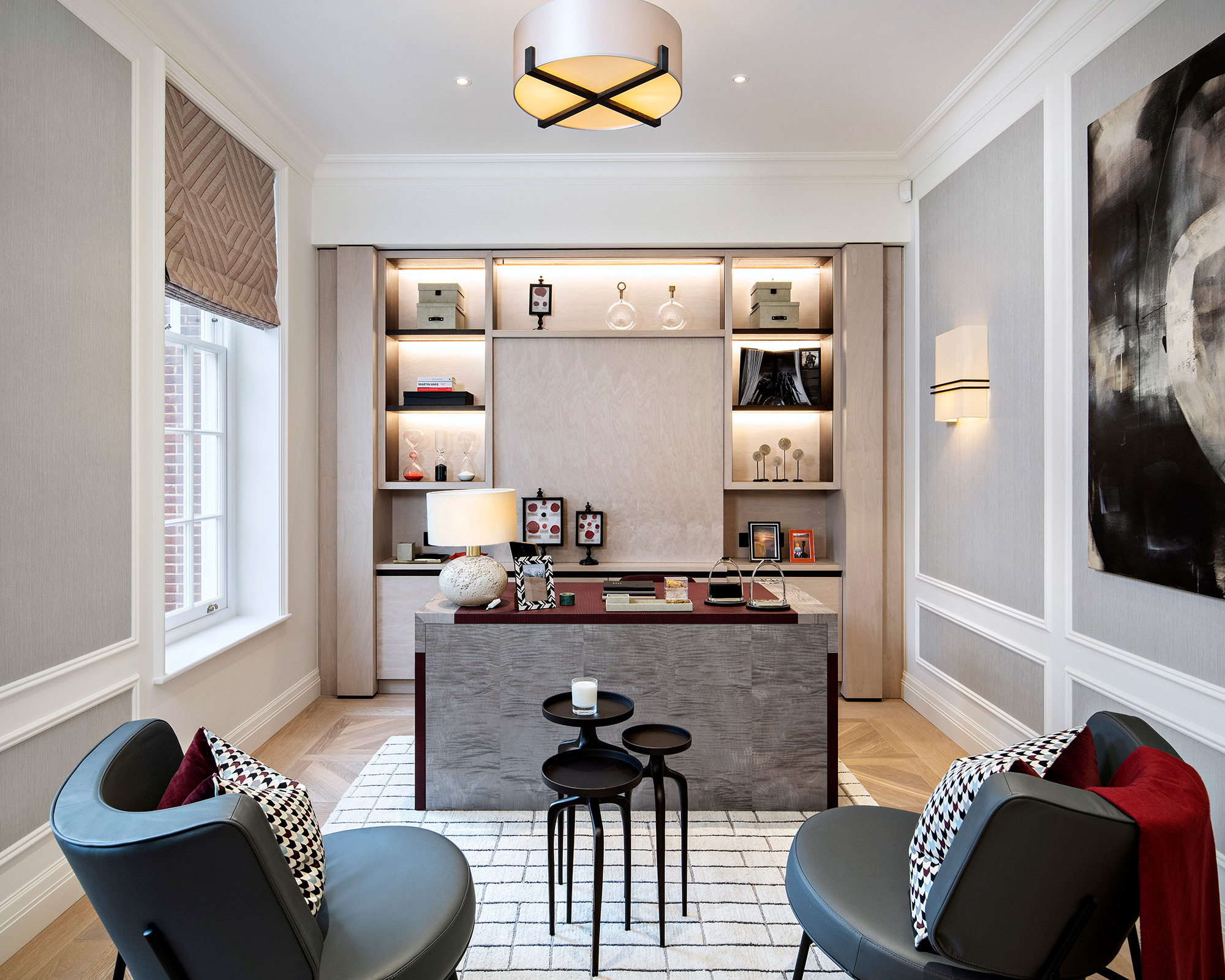The photograph depicts a stylishly decorated living room or office space, captured indoors during the daytime. The room features light gray painted walls with white borders and wainscoting. The focal point is a central desk with a cherry red top and gray metal sides, adorned with a white-shaded lamp, various framed pictures, and other stationary items. Beneath the desk is a visually striking rectangular white rug with dark gray stripes, resembling painted brick.

To either side of the desk are gray chairs, each accented with red throw blankets and pillows—red-backed with a white front decorated with black squares. Adjacent to these are black, three-layer tables, one of which holds a scented candle. Light brown wood parquet flooring extends across the room, adding warmth to the space.

The room is well-lit with a modern chandelier overhead featuring an amber light, additional wall sconces to the right, and a recessed, lighted shelving unit on the back wall. This unit is filled with various objects such as boxes, figurines, and framed pictures or photographs. A large black and silver painting also adorns the right wall. To the left side, a recessed window with grey curtains and brown blinds offers a view of a brick building outside. The window itself is framed with white grids, enhancing its classic look.

Overall, the space boasts a harmonious blend of modern and classic decor elements, making it both functional and visually appealing.